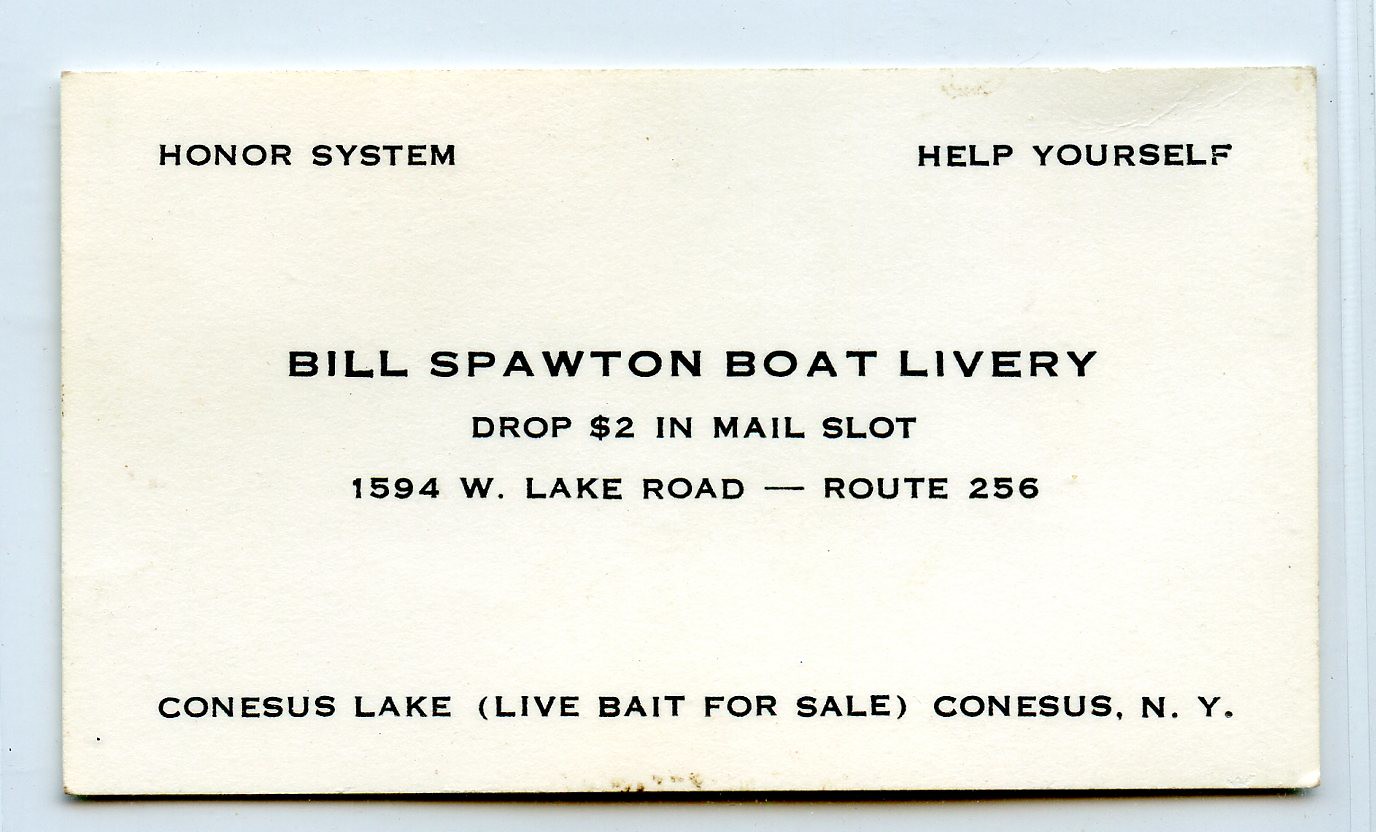This rectangular image, predominantly longer horizontally, features a slightly dirty white postcard with visible spots, marks, and scuffs, set against a very light blue background. The postcard contains black text. In the upper left corner, it reads "HONOR SYSTEM," and in the upper right, it says "HELP YOURSELF." Centered in larger text is "Bill Spaughton Boat Livery." Below that, the text instructs, "Drop $2 in Mail Slot," followed by the address "1594 Westlake Road, Route 256." The card further notes at the bottom, "Can Kinesis Lake (Live Bait for Sale), Kinesis, New York." This postcard advertises bait available for sale on an honor system basis.